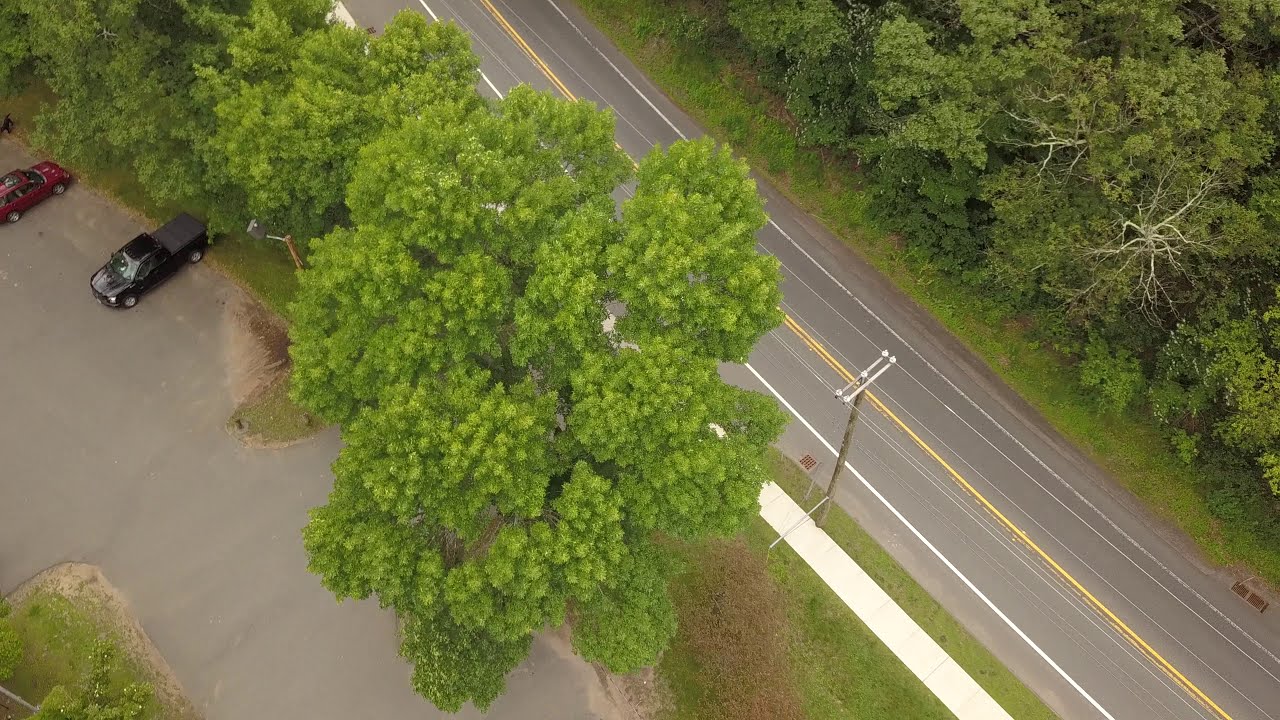This is an aerial daytime image showcasing a tranquil roadside scene. Dominating the lower right corner and extending diagonally upward to the center top is a two-lane road with a solid yellow line in the middle and solid white lines along the edges. The road, devoid of traffic, features shoulder areas for potential parking on both sides. Adjacent to the road on the right is a sidewalk bordered by a power pole with connecting lines. This sidewalk is set amidst a row of tall evergreen trees and lush bushes, filling the upper right corner with vibrant greenery.

On the left side of the road lies a concrete area serving as an informal parking lot, distinguished by the absence of marked spaces. Here, two vehicles are parked: a black pickup truck and a red car, possibly a hatchback or sedan. Adding to the scenic greenery, another cluster of trees occupies this left side of the image, interspersed between the parking area and the road. The upper left portion mirrors the verdant scene with more trees and a grassy patch, completing the serene and natural atmosphere captured in this horizontally aligned rectangular picture.